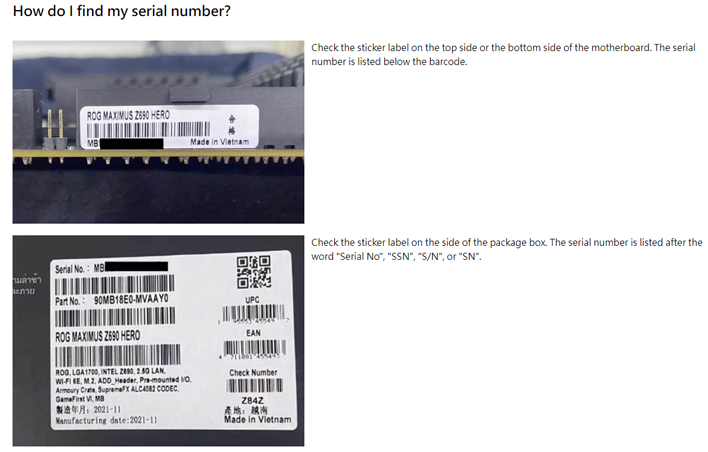The webpage is designed to guide users on locating the serial number of their device. The page lacks a search bar and has minimal identifying details, set against a plain white background with primarily black text.

In the upper left corner, a bold heading reads, "How do I find my serial number?" Directly underneath, there is an image depicting a piece of hardware which could be from a computer, laptop, or possibly a smartphone – some form of technology. This hardware image prominently displays a SKU, the product name, and a serial number. 

To the right of the image, a detailed instruction box explains: "Check the sticker label on the top side or the bottom side of the motherboard. The serial number is listed below the barcode." 

Further down, additional guidance specifies: "Check the sticker label on the side of the package box. The serial number is listed after the word 'Serial No.' 'SSN,' 'S/N,' or 'SN.'" 

Beneath the main image, another section illustrates how a user would locate the serial number following the given instructions.